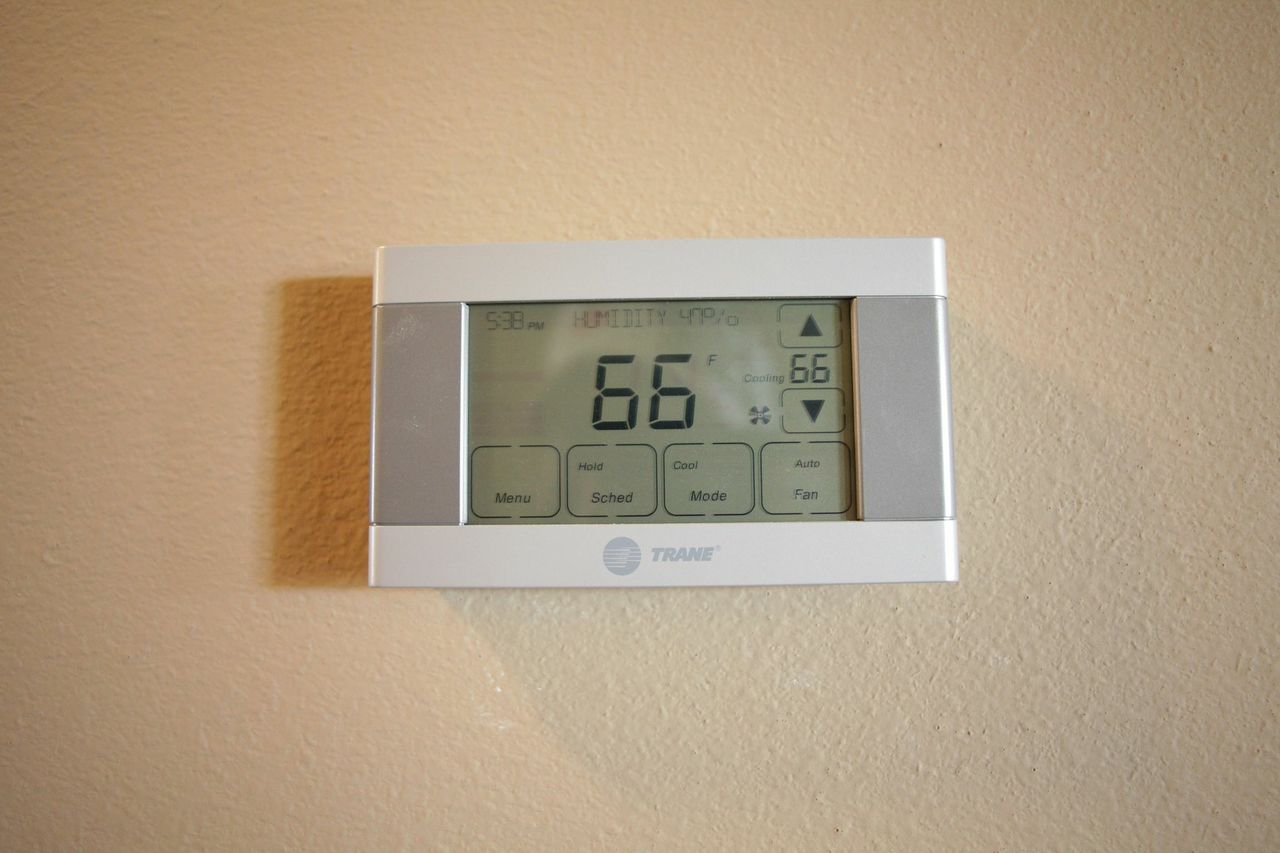A detailed image captures a textured stucco wall with an off-white color subtly tinged with peach. At the center of the photograph, a prominently displayed thermostat becomes the focal point. The well-lit scene highlights the plastic device, which features a sleek gray and silver cover. The thermostat brand, "Trane," is clearly marked at the bottom alongside a distinctive circle logo with a white streak. 

The illuminated display of the thermostat glows with a tan hue, revealing various details: the current temperature is set at 66 degrees Fahrenheit, the time is 5:38 p.m., and the humidity level is 47%. The interface, which appears to be a touchscreen, includes accessible options such as menu, schedule, mode, and fan settings. To the right side, up and down arrows indicate the ability to adjust the temperature, currently fixed at 66 degrees. The device’s fan is set to auto, the mode is on cool, and the schedule feature is on hold. Subtle shadows cast by the lighting add depth and dimension to the scene.